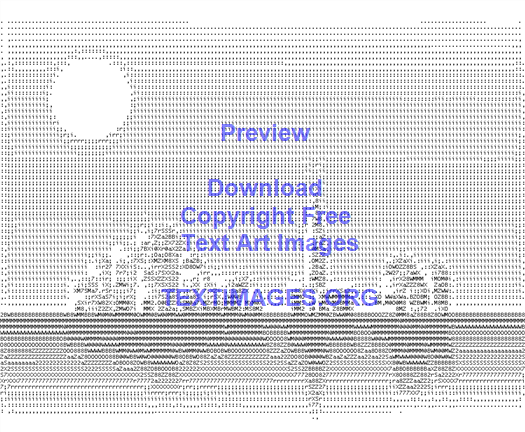This black-and-white digital artwork from textimages.org is created with dot matrix text characters, forming an intricate grayscale landscape that appears to be a city skyline or mountain range with a cactus. The scene features a moon or sun in the upper left corner, casting a shadow on a lake below. Overlaid on the image is lilac or medium purple text that reads "Preview, download, copyright-free text art images," followed by the web address "textimages.org." The text is centrally positioned and spans multiple lines, blending seamlessly with the old schematic or line-drawn aesthetic of the image.